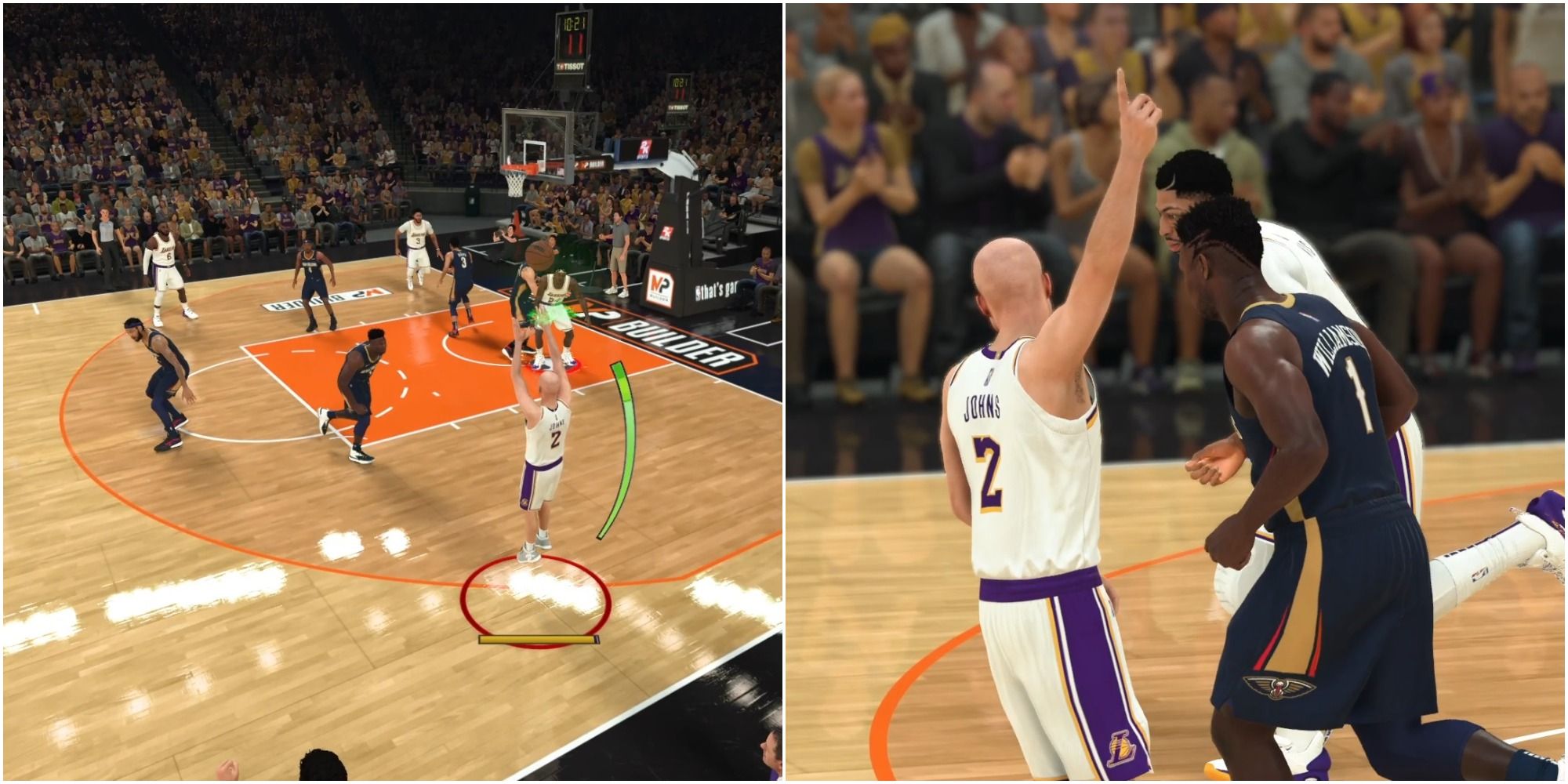The image consists of two square pictures side-by-side, separated by a very thin vertical line, depicting scenes from a basketball video game. In the left picture, taken from a spectator's viewpoint, a player dressed in white with a distinctive purple stripe down his shorts is caught in mid-jump, about to take a shot from beyond the three-point line. This player has been highlighted with a red circle around him. Other players on the court are either wearing white or navy blue with gold trim. The image captures the dynamic atmosphere with the fans in the stands visible, albeit blurry. The right picture offers a closer view of the same player, with 'Johns 2' visible on the back of his jersey and his bald head distinct. Celebrating with one arm up and finger pointing, he stands next to another player in navy blue, with additional players running by. Both images create a vivid, detailed portrayal of the in-game action and the surrounding excitement.